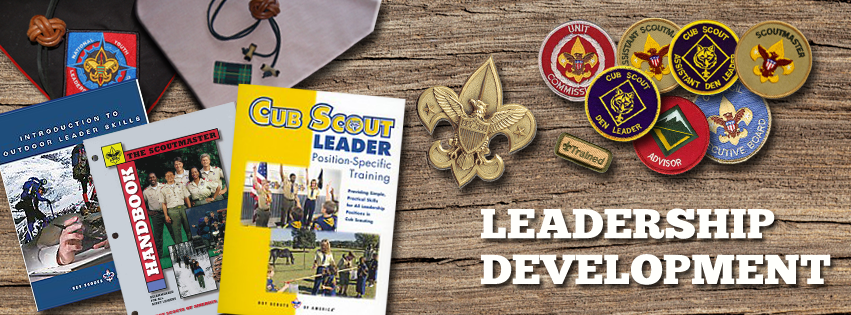This horizontal, rectangular image serves as an advertisement or informational poster for the Cub Scouts, prominently featuring leadership development resources. The left side of the image displays three staggered books: a yellow and blue book titled "Cub Scout Leader Position Specific Training" with its title in bold bubble letters, a grey and red "The Scoutmaster Handbook" featuring a photo of Cub Scouts, and a blue "Introduction to Outdoor Leader Skills." On the right side, large white text reads "Leadership Development," accompanied by the Cub Scout trefoil logo with an eagle. Above this text are seven Cub Scout badges representing various roles such as Den Leader, Advisor, Executive Board, Scoutmaster, Assistant Den Leader, Assistant Scoutmaster, and Unit Commissioner. All elements rest on a wood grain background, enriching the image with a rustic feel.